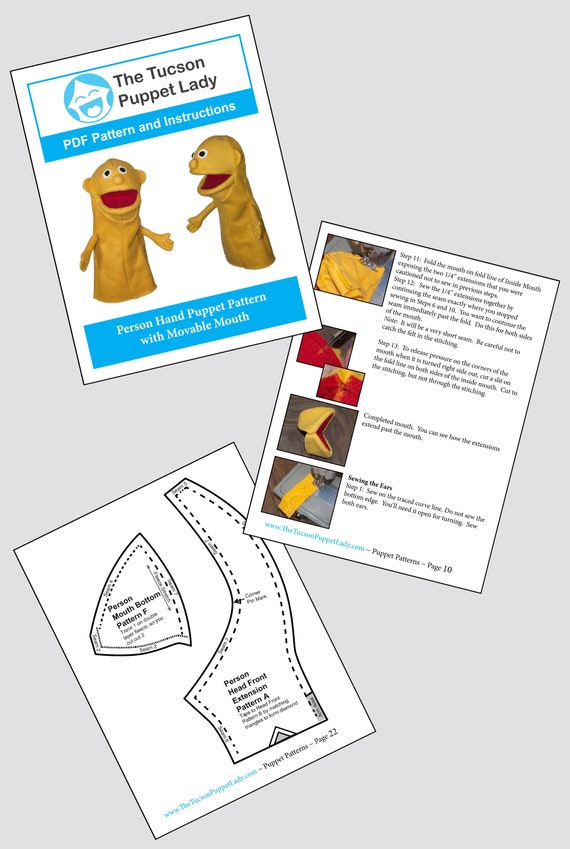In this image, we see a collection of three documents laid out on a light gray surface. The first document, positioned at the top, features the title "The Tucson Puppet Lady" in black text. Below this, a blue banner with white text reads "PDF Pattern and Instructions." Further down, another blue rectangle contains the text "Person Hand Puppet Pattern with Movable Mouth." Between these banners, two views of a bright yellow puppet with a red mouth and black and white eyes are displayed — one from the front and one from the side. The puppet has a circular nose, semicircular ears, and a rectangular body with outstretched yellow arms.

The second document, placed at a diagonal angle to the right, contains a detailed set of instructions for creating the puppet. It features a series of small images and accompanying text, though the font is too small to discern the specifics. The images appear to illustrate various stages of the puppet-making process, showcasing colors like yellow, red, and brown.

The third document, laid out diagonally to the left, is a black-and-white pattern guide for cutting out shapes needed to assemble the puppet. This guide includes labeled diagrams and spotted lines along the borders of the shapes, which include a triangle and a hook-like figure. All three documents collectively provide a comprehensive guide to creating a hand puppet, from visual references to detailed instructions and pattern templates. The grey backdrop complements the white paper, making the documents and their colorful elements stand out clearly.